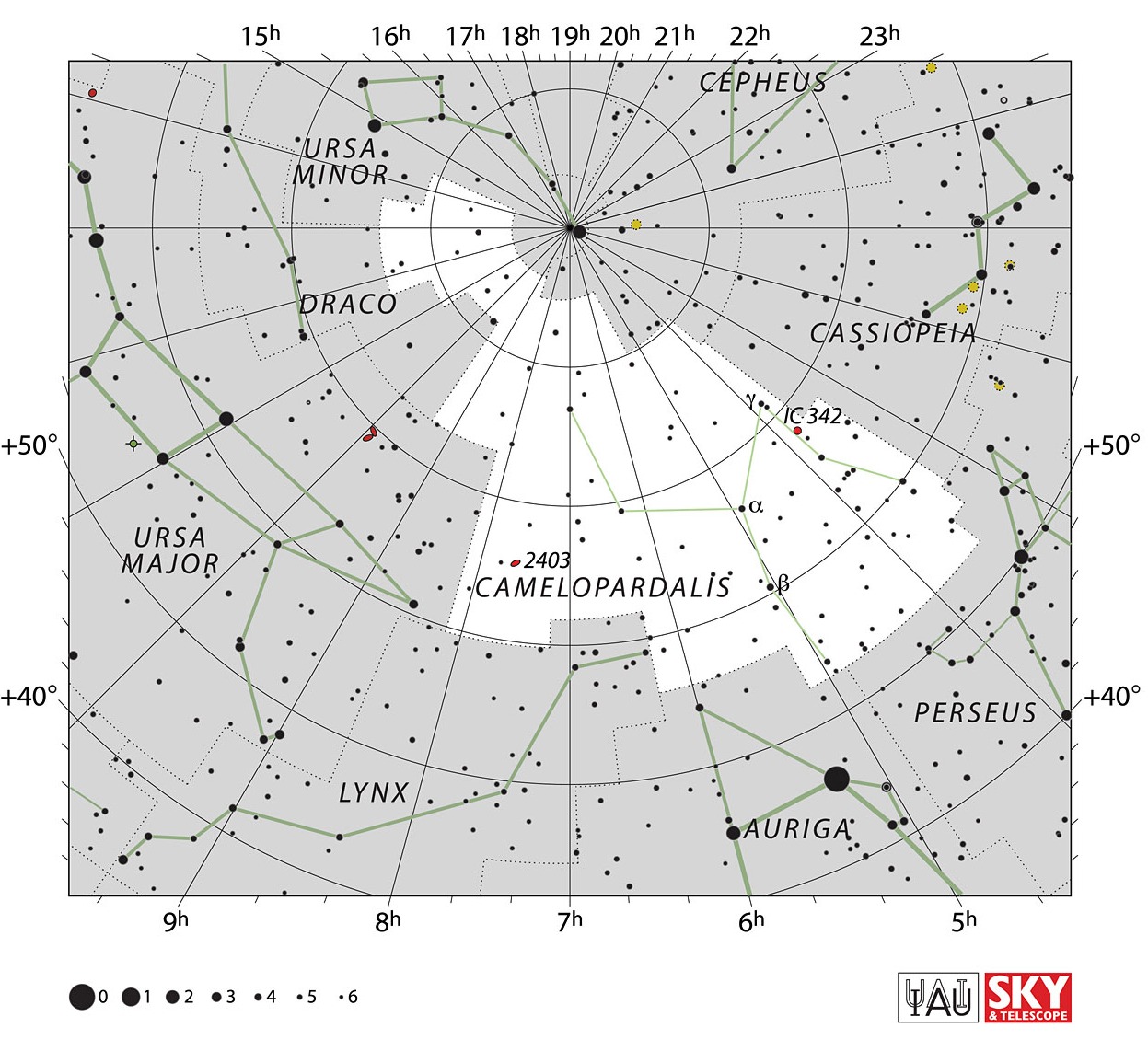This is a detailed star map diagram illustrating various constellations in the night sky, including Cassiopeia, Cepheus, Ursa Minor, Draco, Ursa Major, Lynx, Perseus, Auriga, and Camelopardalis. The map is organized on a grid with coordinates: at the top, it features sequential hour markers from 15H to 23H, while the bottom ranges from 5H to 9H. Both the left and right sides are marked with latitude indicators at plus 40 and plus 50 degrees. The map contains numerous dots representing stars, many of which are connected by lines to form constellation patterns. The background features a color palette of gray, white, black, and red. Annotations include "IAU Sky and Telescope" on the bottom right corner. The overall style is a clear and precise star map designed for detailed celestial observation.